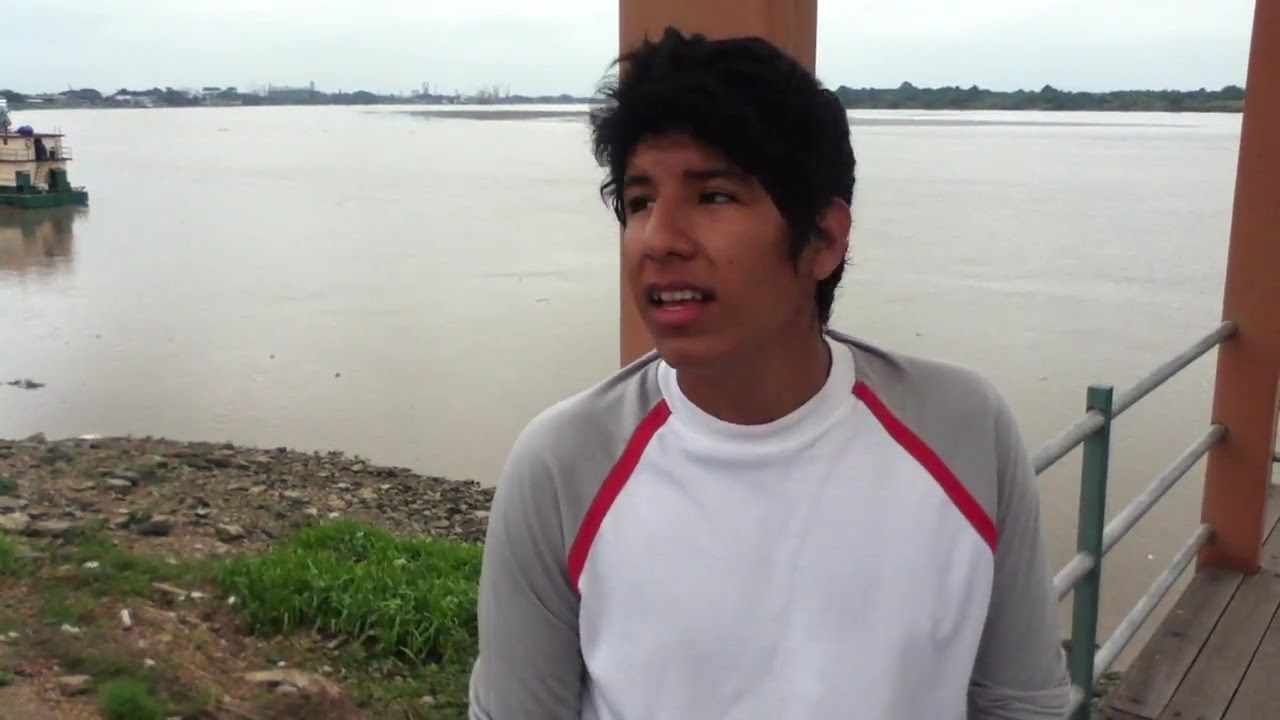A color photograph in landscape orientation captures a young, dark-haired male, estimated to be between 15 to 20 years old, from head to elbows. He gazes to his right, and wears a distinctive shirt featuring a white front with gray sleeves and red stripes running from neck to armpits. Standing on a wooden pier or dock with a railing, he is positioned in front of a large body of water, possibly a lake or bay. The shoreline is visible to his right, characterized by a mix of stones, grass, and a small area of rocky terrain. In the top left of the image, a portion of a boat or ferry is seen, suggesting a serene, somewhat industrial or urban lakeside setting. The distant background reveals another shoreline and an overcast sky, adding to the overall calm ambiance of the scene.